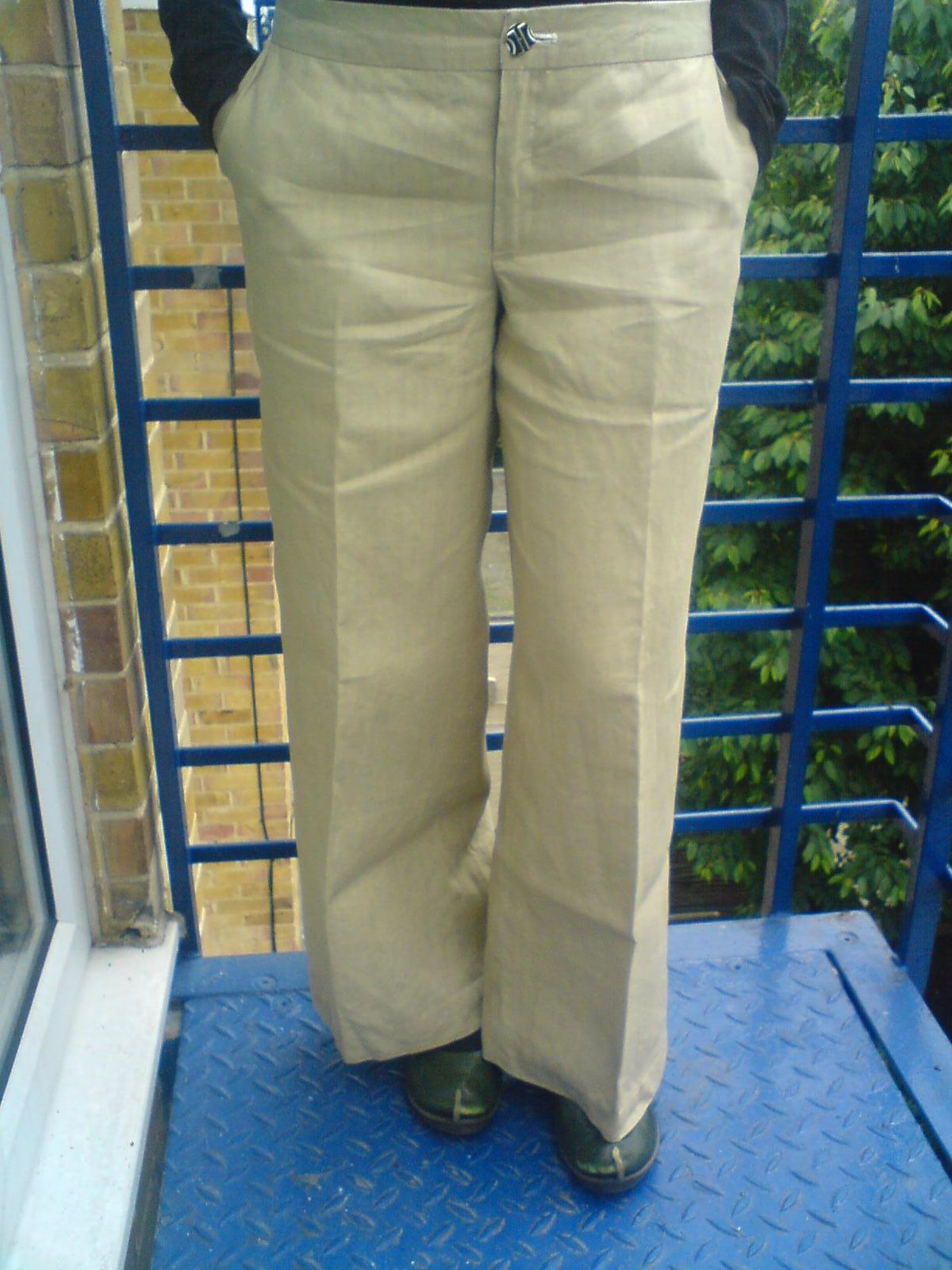The image is a color photograph of a person standing on a blue metal platform, which resembles a fire escape or balcony. The platform has a blue metal railing and a metal grid flooring, attached to a white frame with a glass center, possibly a door or window frame. The person is visible only from the waist down, wearing khaki-colored bell-bottom pants with a silver button shaped like an 'H.' Their hands are in their pockets, partially revealing the sleeves of their long black shirt. They are also wearing green shoes with grey soles. In the background, there’s a tree almost as tall as the platform, covered in green leaves, indicating that the setting is outdoors with ample natural light. The left side of the image features part of a building wall, likely brick, adding to the outdoor ambiance.